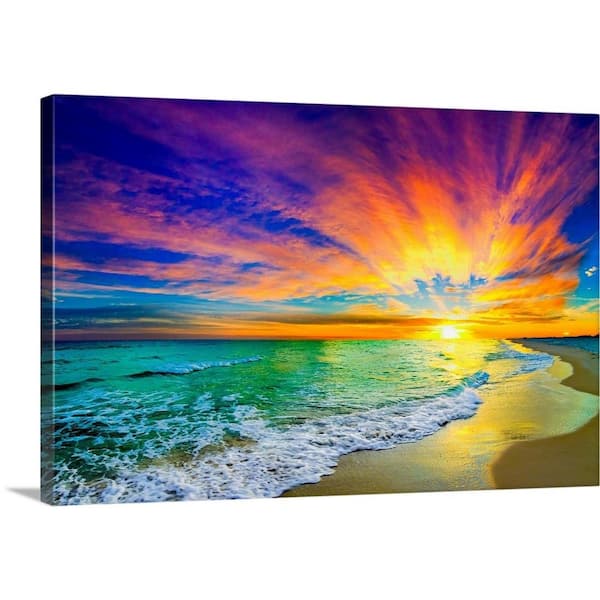This image captures a vibrant sunset over a beach, printed on canvas that has been stretched and wrapped around a solid frame, giving it a 3D appearance. The top half of the image showcases an intensely colorful sky, with an azure blue backdrop featuring wispy and thick clouds reflecting shades of pink, orange, yellow, deep amber, and lavender, suggesting the application of a filter. The setting sun casts a golden light, creating striking sunset streaks. Below the sky, the turquoise-colored ocean with its foamy waves stretches diagonally from the bottom left to the upper right, leading to a sandy beach on the lower right. The beach features wet sand reflecting the sunlight and transitioning to drier sand. This intricate setup, with the photo seemingly folded around the frame, adds depth, making it nearly infinite in visual appeal. The shadows behind the canvas add to the 3D effect, enhancing the overall realism of this enchanting coastal landscape.